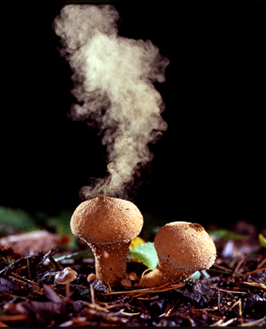This image depicts two brownish-beige mushrooms situated on a forest floor covered in natural debris such as leaves and sticks. Both mushrooms have a solid, wide base, and the one on the left is taller and points straight up, while the one on the right tilts to the side. The surroundings are dark with a pitch-black background, suggesting the photo was taken at nighttime or in a controlled environment like a terrarium, lit by a bright, direct light source from the upper right. Intriguingly, white smoke rises behind the left mushroom, giving the impression of spore release, although some believe this smoke might be artificially added or edited into the image. The scene is rich with natural details and has an eerie, mystical quality due to the combination of lighting and the curious presence of smoke.